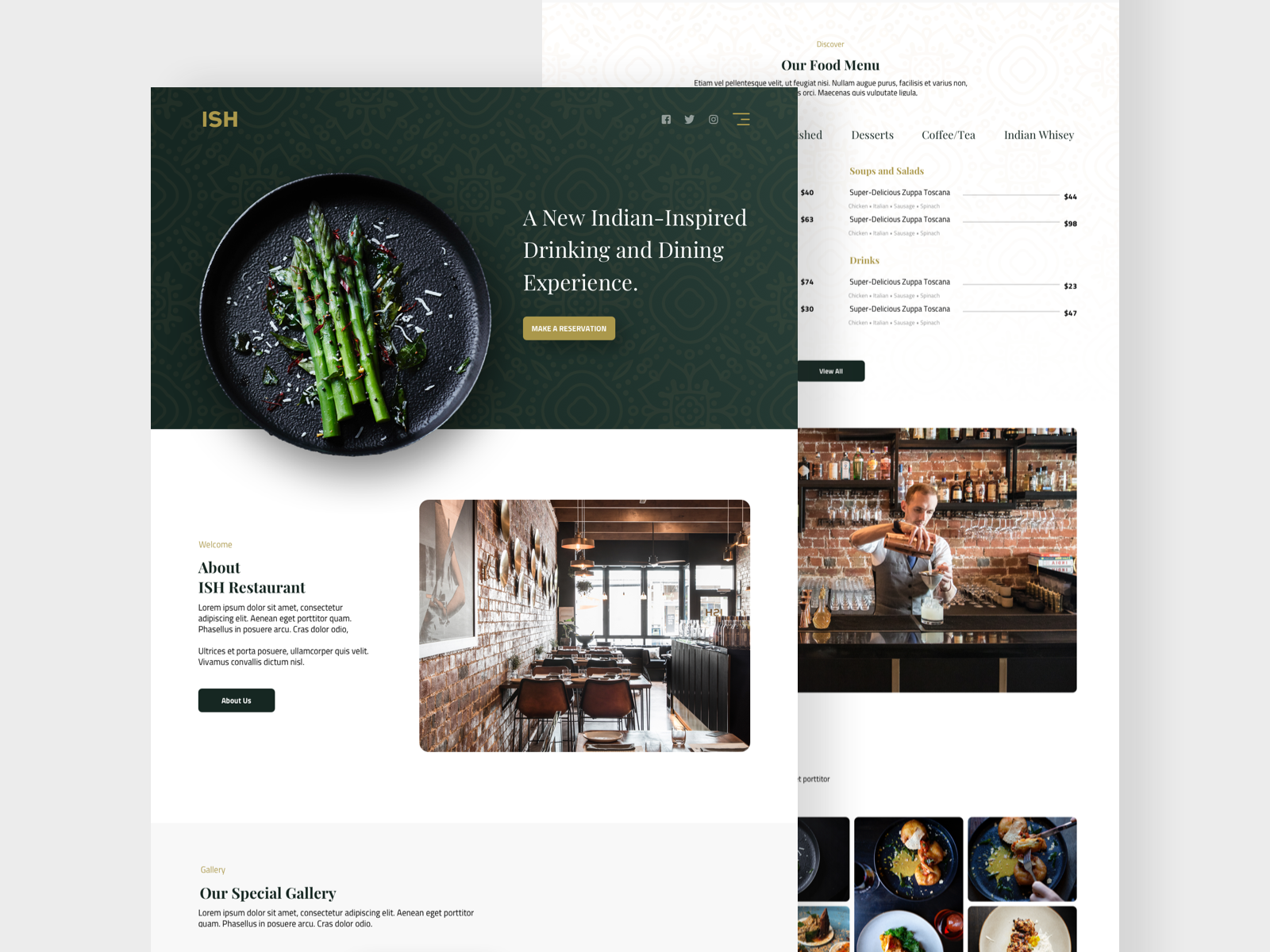The image depicts a vibrant promotional webpage for a dining establishment named ISH. Dominating the top section of the page is a green box featuring an enticing visual of asparagus spears sizzling on a skillet, interspersed with delicate shavings. The centered bundle of five or six asparagus stalks captures the simplicity and elegance of the dish. 

To the right of this culinary image, a bold white text announces: "A New Indian Inspired Drinking and Dining Experience," inviting potential patrons to delve into the innovative cuisine. Below this announcement, a call-to-action button labeled "Make a Reservation" beckons visitors to secure their dining experience.

Above the announcement, social media icons for Facebook, Twitter, and Instagram encourage users to follow the restaurant's updates and engage with its online presence. Moving down the page, another section titled "About the Restaurant, ISH" provides a concise introduction to the restaurant, complemented by a button labeled "About Us" for more detailed information.

Adjacent to this description is a photograph of the restaurant’s interior, highlighting a modern aesthetic with a cozy ambiance. The image showcases a brick wall adorned with hanging brass lights, illuminating three tables, each flanked by pairs of chairs. A windowed divider on the right leads the eye towards the far corners of the establishment.

Further down, the section titled "Our Special Gallery" offers an overview of ISH's culinary offerings, accentuated by various images. The food menu is prominently featured, listing items such as desserts, coffees, whiskey, and soups and salads, along with their prices and special deals like two drinks for the price of one.

A dynamic image of a bartender skillfully pouring a drink adds a personal touch, alongside an assortment of images showcasing a variety of food, including pastries, solidifying ISH's reputation for diverse and appealing menu options.

This detailed and visually engaging webpage encapsulates the essence of ISH, promising a unique and contemporary dining experience deeply rooted in Indian-inspired flavors.